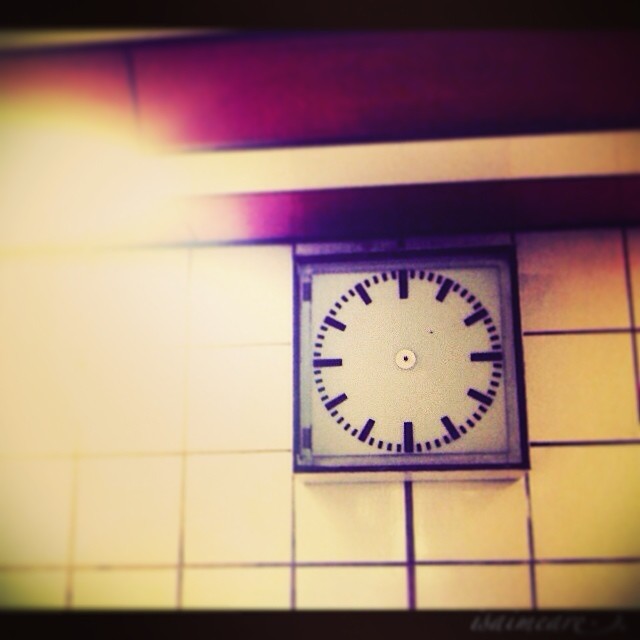The image depicts a somewhat overexposed view of a clock mounted on a wall, marked by a pronounced light glare predominantly on the left-hand side. The wall features a combination of brown wood panels and a white stripe toward the top, transitioning into white subway tiles with black grout below. This intricate tiling extends vertically and horizontally. The clock itself is square with black edges and a light silver or white clock face. It’s designed with black dashes indicating the hours and smaller dashes representing the minutes. The clock, however, lacks its hands. There are noticeable shadows and a red curved ceiling above a white ledge. The image also has an element of blurred text toward the bottom right. Yellow and orange light hues cast from the left further highlight the yellowish-orange color of the wall.